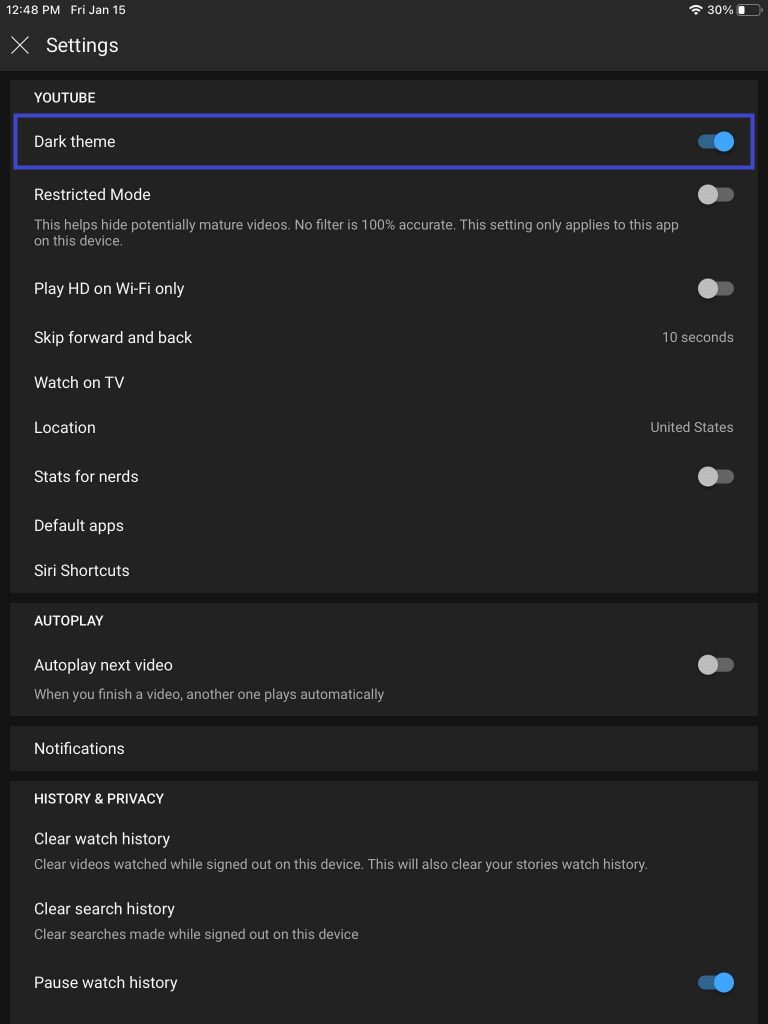This screenshot captures the settings interface of the YouTube mobile application. The top of the screen displays standard cell phone icons, such as signal strength, battery level, and time, positioned at the upper corners. Just beneath the date on the left-hand side, the word "Settings" appears in bold white font. Directly below this label, a black bar stretches horizontally across the screen, serving as a divider.

The word "YouTube" is prominently displayed on the left side in uppercase white letters. The first option listed under this heading is "Dark theme," which features a blue rectangular outline and is toggled on. Following this, "Restricted mode" is listed and currently toggled off. The "Play HD on Wi-Fi only" option is also shown but toggled off.

The screen continues with the "Skip forward and back" setting set at 10 seconds. This is followed by "Watch on TV" and then the "Location" setting, which is configured to the United States. Lastly, the "Stats for nerds" option is listed at the bottom and toggled off.

The overall design is sleek, with clearly delineated sections and toggles for each setting, making navigation intuitive and user-friendly.